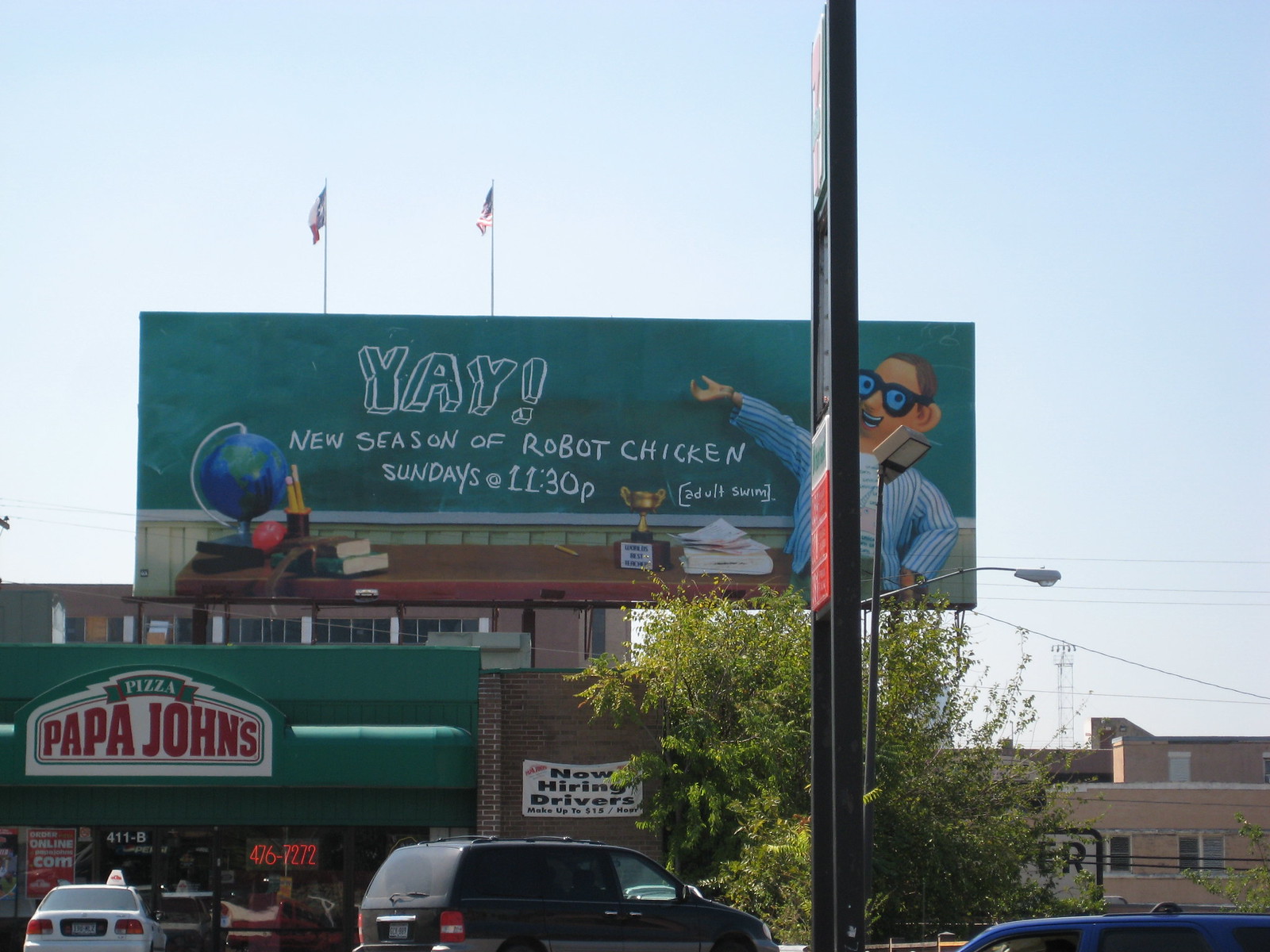A vibrant photograph capturing a bustling parking lot outside a Papa John’s restaurant. Several cars are parked in the foreground, though their lower halves are truncated by the frame. The Papa John’s sign, prominently displayed, features the iconic logo with "Papa John's" and "Pizza" inscribed at the top. Beneath it, a large banner announces “Now Hiring Drivers,” indicating the restaurant's need for delivery personnel. 

Above the restaurant, a billboard promotes the new season of the animated comedy show “Robot Chicken,” airing Sundays at 11:30 p.m. on Adult Swim, complete with a colorful cartoon image from the show. In the background behind the billboard, two small flags, likely American, can be seen fluttering in the wind. Additional elements such as nearby buildings, a street lamp, and overhead wires add depth to this urban scene.